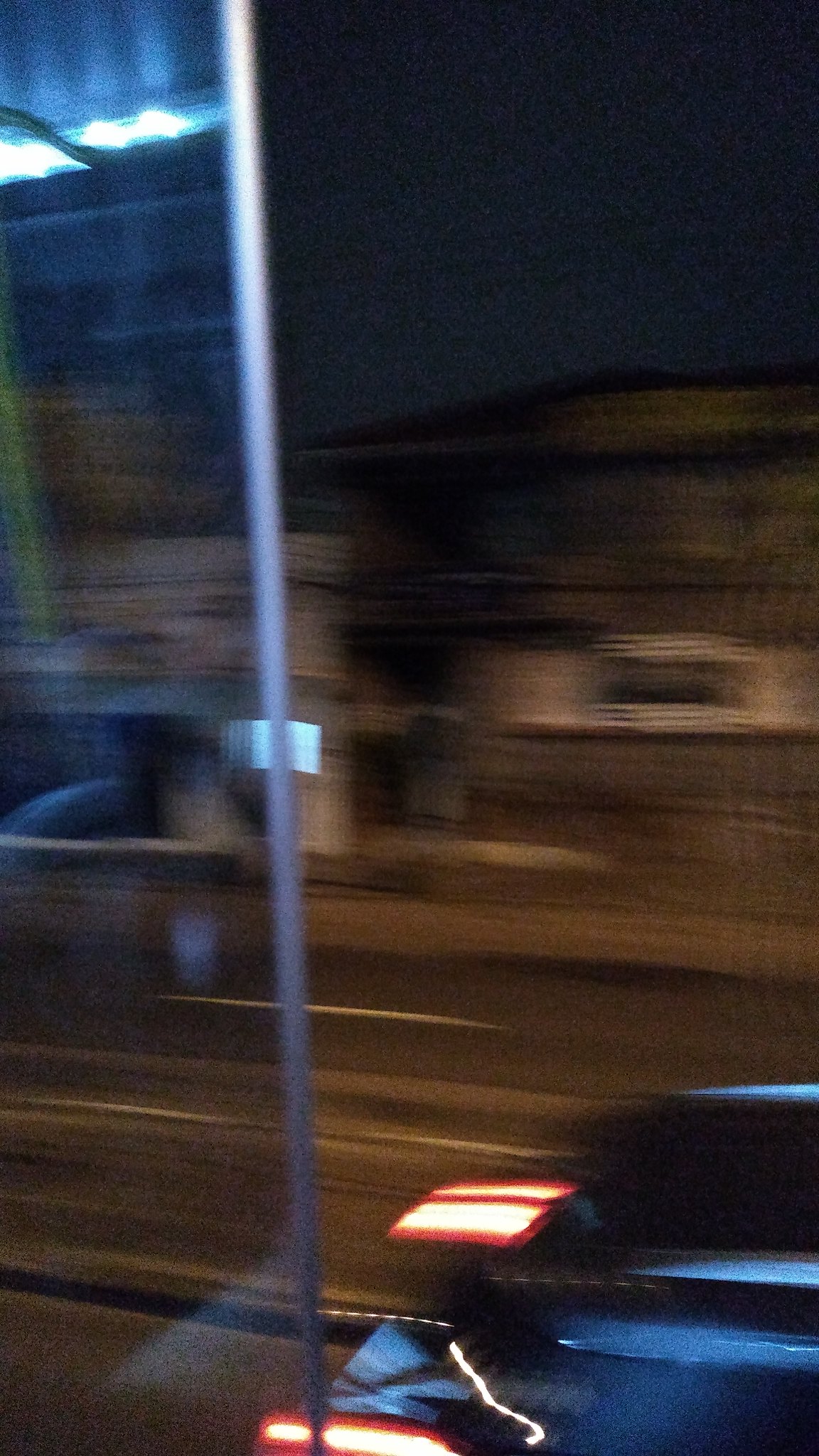The image, likely taken with a phone due to its vertical orientation, offers a first-person perspective from inside a home, looking out through an open glass patio door. The scene is captured at night, and the picture's blurriness suggests the photographer was in motion. To the left of the frame, the glass door is visible, pushed open. Through the opening, the street outside is revealed, with the lights of a blue truck and a white car in motion, each traveling in different lanes. Across the street, a white house with lights on its patio can be seen, though reflections on the glass and the general blur obscure some details. The dark night sky forms the backdrop, enhancing the nighttime atmosphere.